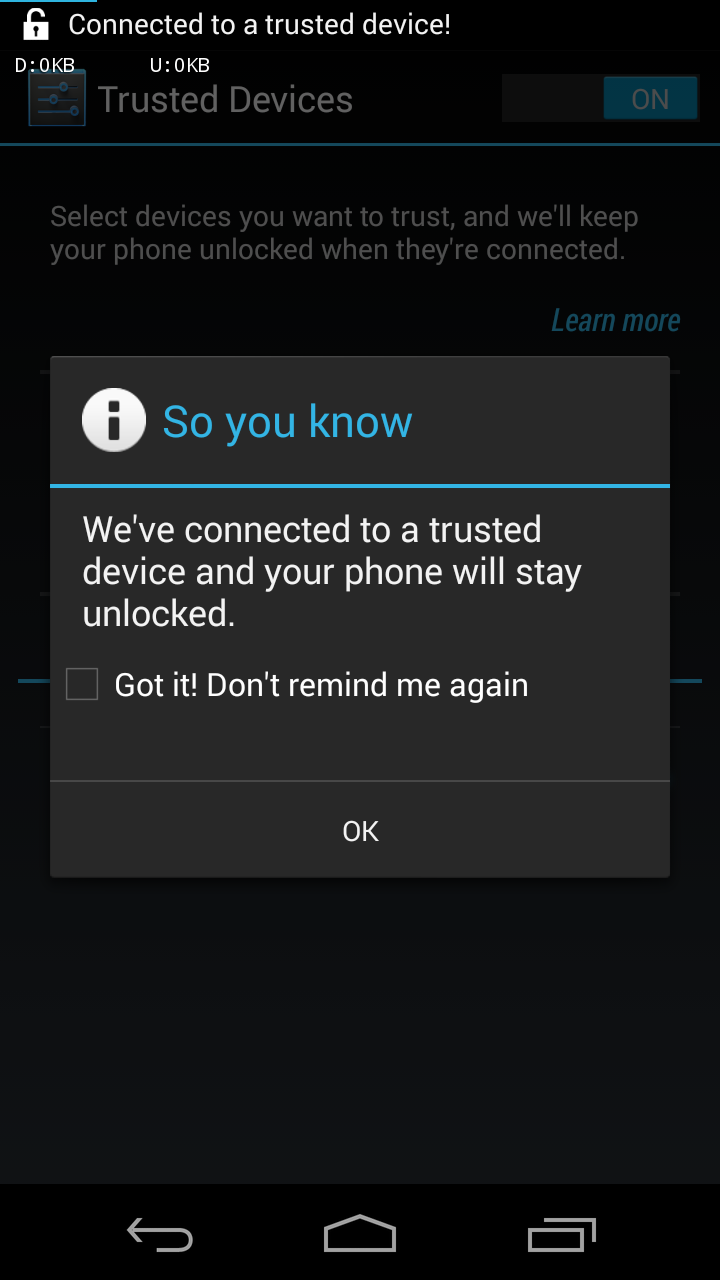**Detailed Caption:**

This image is a screenshot from a smartphone displayed vertically on the screen. In the upper left-hand corner, a white lock symbol is visible, indicating that the lock is unlocked. Adjacent to this symbol, the text reads "Connected to a trusted device" in white letters. Immediately below this message, the data usage indicators show "D: 0 KB" and "U: 0 KB," also in white text. Further down, in faded letters, it states "Trusted devices."

A blue horizontal line spans across the screen, followed by the instruction, "Select devices you want to trust and will keep your phone unlocked when you're connected. Learn more."

Dominating the center of the screen is a pop-out notification box with a black background and a square shape. In the upper left-hand corner of this pop-out, there is a round white icon with the letter "i" in the center, signifying information. Beside this icon, in blue letters, the message "So you know" is displayed. Below this, a horizontal blue line divides the content. Underneath the blue line, white text reads, "We've connected to a trusted device and your phone will stay unlocked."

Towards the bottom of the pop-out notification, there is an unchecked checkbox accompanied by the text, "Got it, don't remind me again." At the very bottom center of this pop-up, a button labeled "OK" is visible.

Overall, the screenshot captures a moment on the smartphone where the user is being informed that their device is connected to a recognized and trusted device, which allows it to remain unlocked.